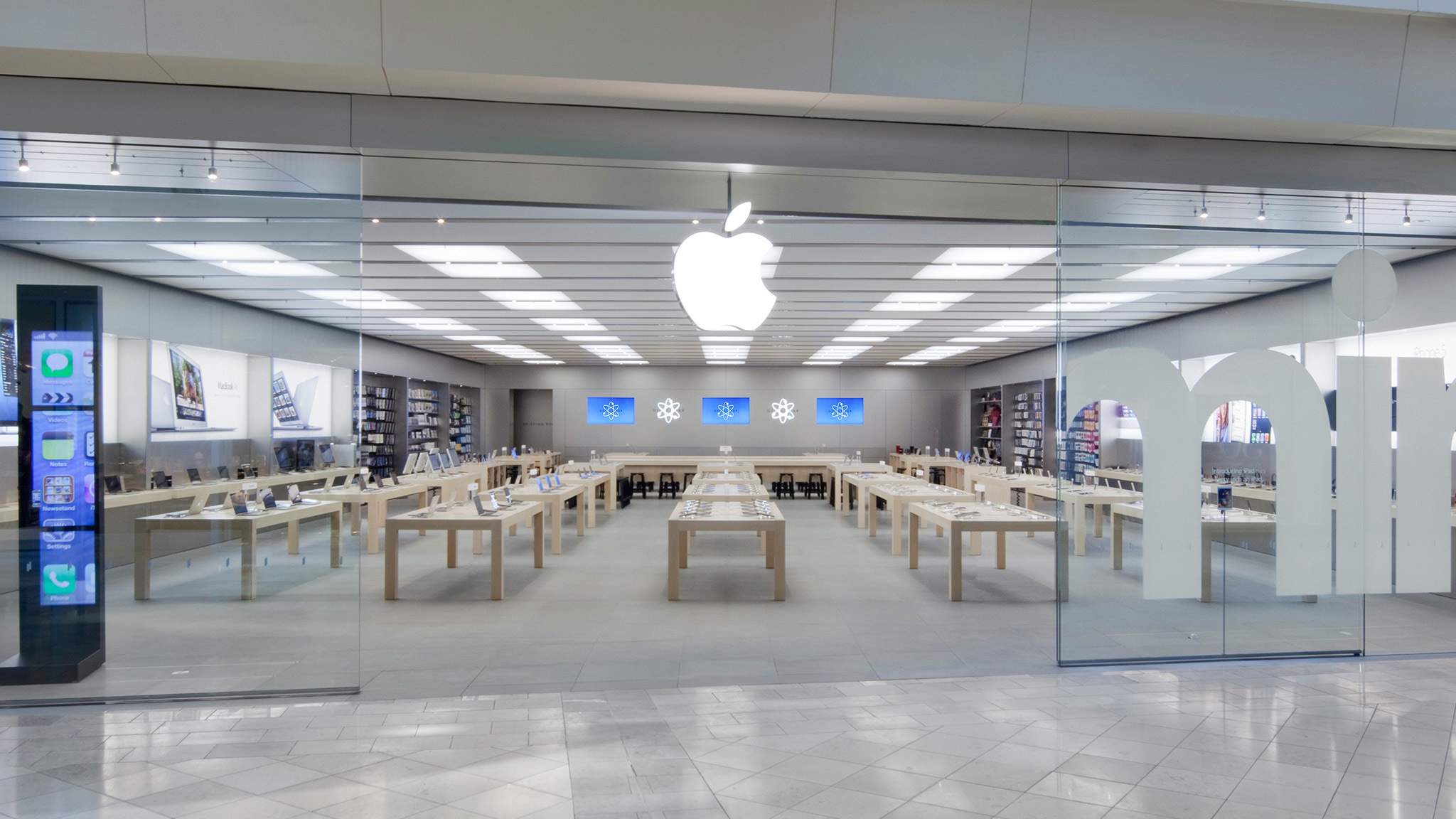A photo captures the exterior of an Apple store located within a mall. The scene is dominated by a pristine, white, and shiny linoleum floor, meticulously laid out in marble tiles. The store’s glass doors are effortlessly open, inviting patrons inside. On the right side of these doors, the partial letters "M-I-L" are visible, hinting at possible signage. Above the entrance, the iconic Apple logo stands prominently. 

Inside the store, five orderly rows of tables display various Apple products. Among these, iPads and iPhones are distinguishable, though no laptops are evident, only monitors and screens. The store’s back wall features two cabinets on each side, potentially housing additional products like phone chargers and covers. Monitors are strategically placed throughout the store, including in the back and the front window on the left. The image captures the sleek, organized atmosphere characteristic of Apple retail spaces.